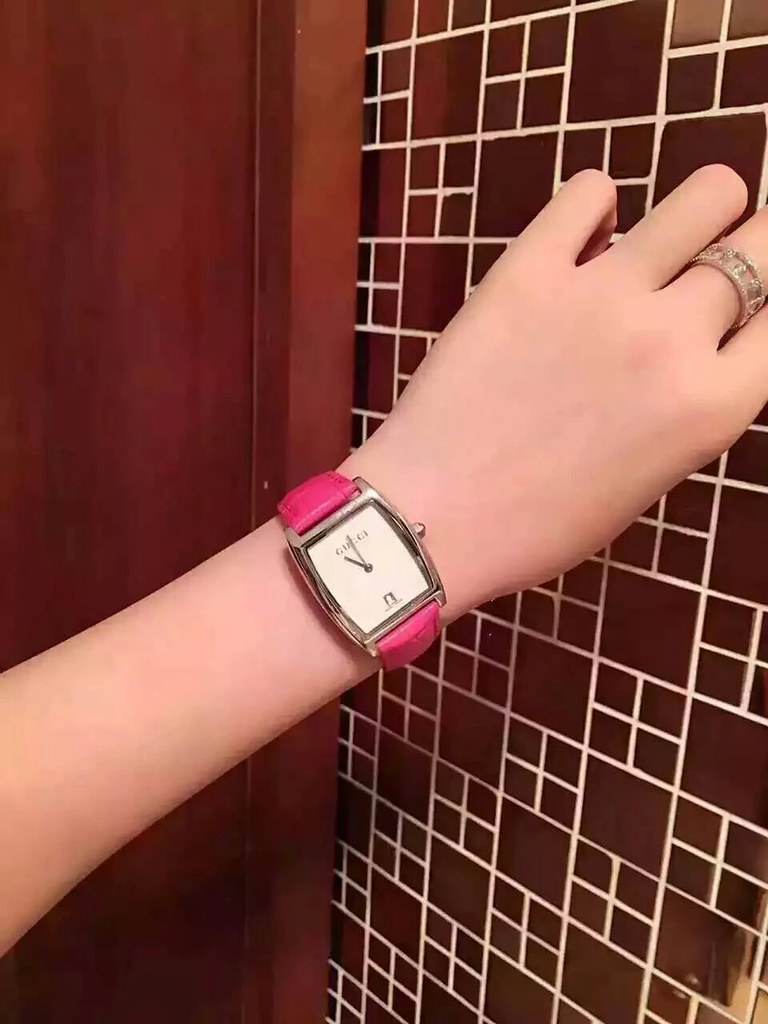The image shows a close-up of a person's thin arm and partially seen hand, extending from the bottom left to the top right of the frame against a background of brown tile and a wooden door frame. The focal point is a striking pink Gucci watch with a vintage aesthetic, featuring a squared, white face with silver accents and a shiny, crocodile-embossed leather strap. Additionally, the individual, presumed to be female, is wearing a distinctive silver crisscross ring on her middle finger, adorned with costume jewelry-like details. The environment is brightly lit, casting light on the arm and showcasing the texture of the tiles and the wood paneling.